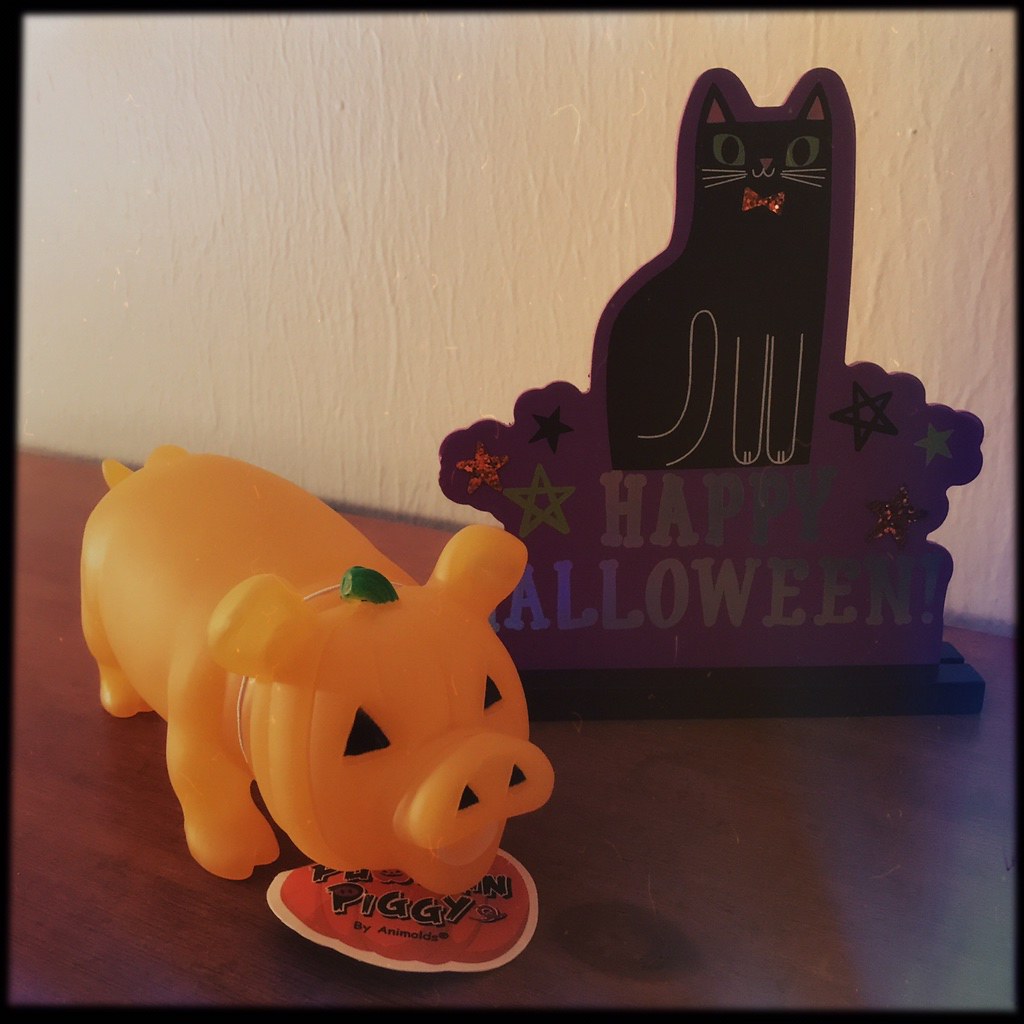The image depicts a scene with Halloween-themed decorations set against a creamy stucco-textured wall. The surface they rest on is a reddish-brown table or counter, where the wood grain and a knot are visible. On the left, there is an orange piglet resembling a jack-o'-lantern, complete with triangle eyes, nostrils, and a green stem-like part on its head. A tag beneath it features the word "piggy." To the right is a cutout sign standing on a black pedestal base with a purple accent. This sign features a whimsically drawn black cat with green eyes, pink ears, white whiskers, and front feet sketched in white chalk. The cat sports an orange bow tie, and its tail curves upward. Beneath the cat, the sign reads "Happy Halloween" accompanied by some stars.